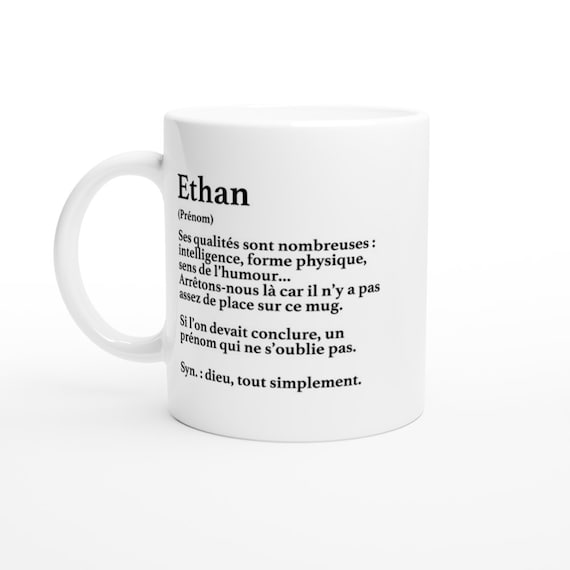The photograph showcases a standard white, 10-ounce coffee mug with a large handle positioned to the left. The name "Ethan" is prominently written in black at the top near the handle. Below "Ethan," there is additional text detailing the qualities and characteristics associated with the name, such as intelligence, good looks, and humor. This description appears to be written in both English and an unidentified foreign language, possibly French. The mug rests on a light-colored surface that blends seamlessly into a grayish-blue or white backdrop, making it challenging to distinguish the exact background.